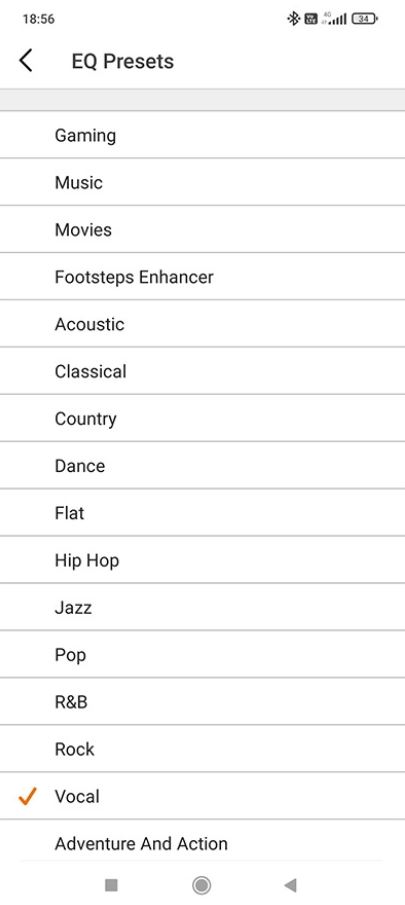This image is a screenshot showcasing a device's interface, captured at 18:56. In the top left corner, the time "18:56" is displayed. Adjacent to the time, a Bluetooth icon is visible, followed by a square icon whose purpose is unclear. Further along are the network signal icon and the battery icon, which also indicates the remaining battery percentage.

Beneath these status icons, the text "EQ presents" is prominently displayed, introducing a comprehensive list of audio equalizer presets tailored for different activities and music genres. The list includes options such as Gaming, Music, Movies, Footsteps, Acoustic, Classical, Country, Dance, Flat, Hip-Hop, Jazz, Pop, R&B, Rock, Vocal, Adventure, and Action. 

At the bottom of the screenshot, there is a navigation bar typical of modern touch-screen devices, showing icons for space, back, and recently opened tabs, allowing users to navigate through their phone's interface easily.